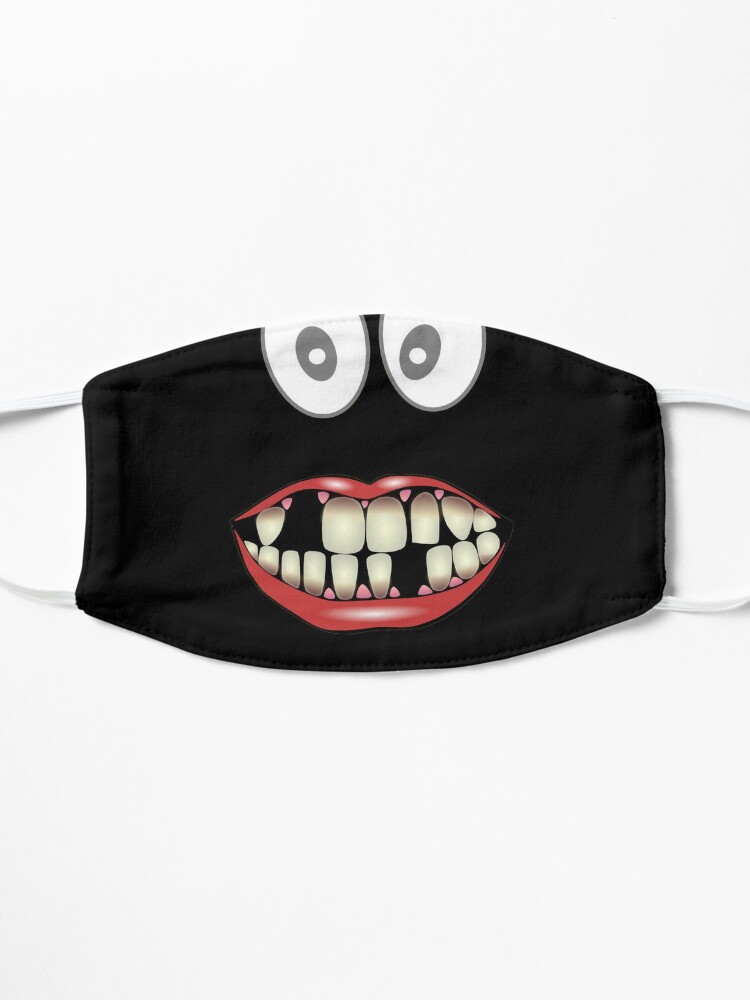This image features a cartoonish face mask designed to cover the nose and mouth, prominently displayed against a plain white backdrop. The mask itself is made from black cloth and features white elastic straps at either side for securing around the ears. The most striking elements of the mask are its playful, whimsical graphics. At the top, the mask has two large, round eyes with gray pupils, giving it a silly, exaggerated facial expression. Below the eyes, there's a wide, open-mouthed smile illustrated with bold red lips. The interior of the mouth reveals a set of yellow-tinted, snaggletooth teeth, with some teeth visibly missing both on the top and bottom rows, enhancing its humorous and quirky appeal. This design, reminiscent of a mischievous or playful character, evokes a lighthearted, jokey vibe, making it clear that the mask is intended as a fun, novelty item rather than a serious face covering.